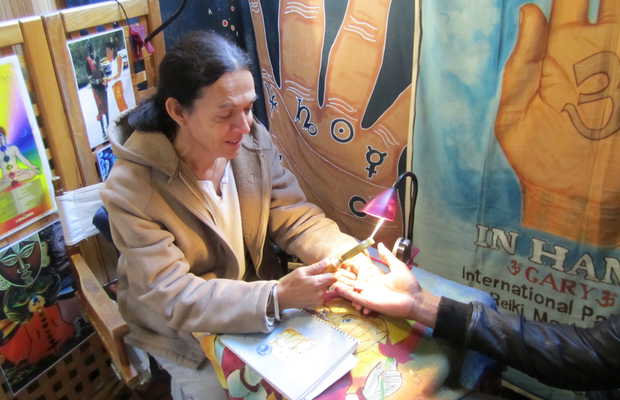The image depicts a woman with black hair tied back in a ponytail, engaged in a detailed palm reading session. She is seated in a small, wooden canvas chair with a white fabric back, leaning forward intently. She wears a tan jacket over a white shirt and holds a magnifying glass in one hand, carefully examining the palm of a person whose body is off-camera, except for their brown leather-jacketed arm. A pink light illuminates the hand being read, which rests on a table also supporting a notebook. The room is adorned with various images and banners, including some featuring hands with zodiac symbols and other esoteric marks. One of the banners reads "In Hand Gary International," but the complete text is not visible. Behind the woman, additional photographs and paintings add to the eclectic, mystical ambiance of the setting.